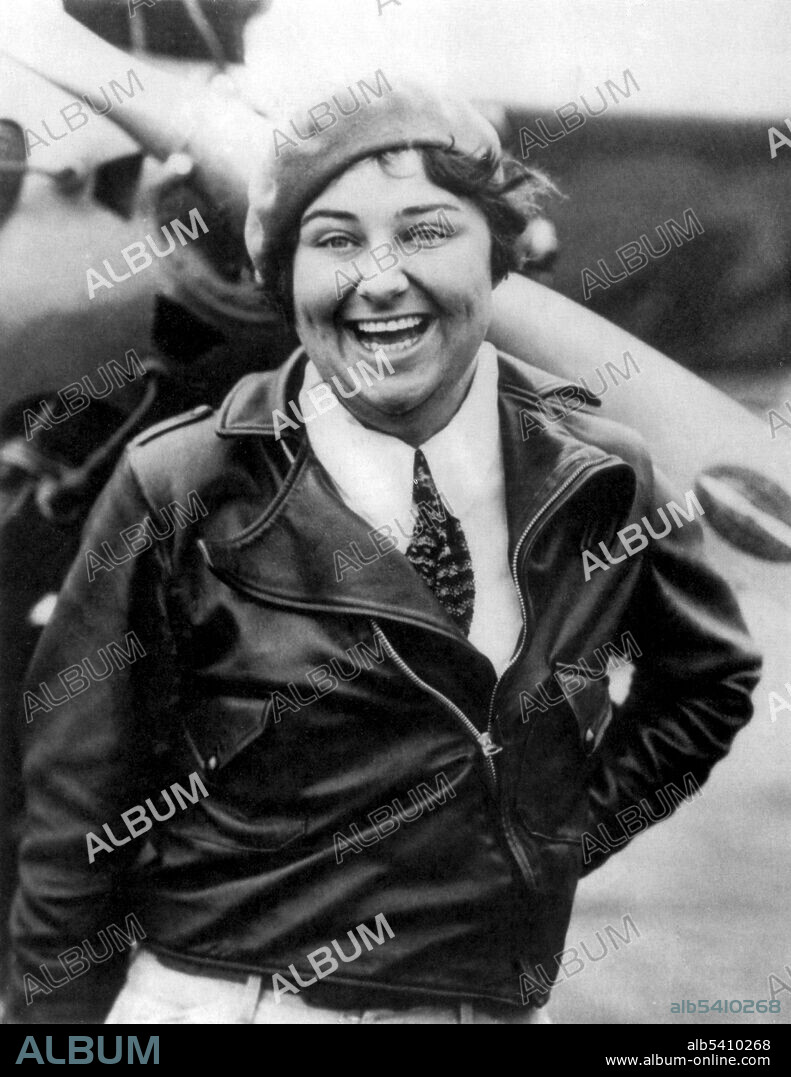This black-and-white photograph captures a joyous woman with short dark hair and a big smile, standing confidently in front of a propeller airplane, likely from the era of iconic aviator Amelia Earhart. The woman, dressed in a black leather jacket with a diagonal zipper, a white shirt, and a necktie, exudes the pioneering spirit of early female aviators. She wears a cap, adding to her pilot-like appearance. The background features a two-bladed propeller, partially blurred but distinct enough to convey the aviation theme. Throughout the image, the word "ALBUM" is repeatedly watermarked in gray, and additional text at the bottom includes "album" in light blue letters and the URL "www.album-online.com". The unique identifier "ALB5410268" also appears in blue and white at the bottom right, reinforcing the album's branding.